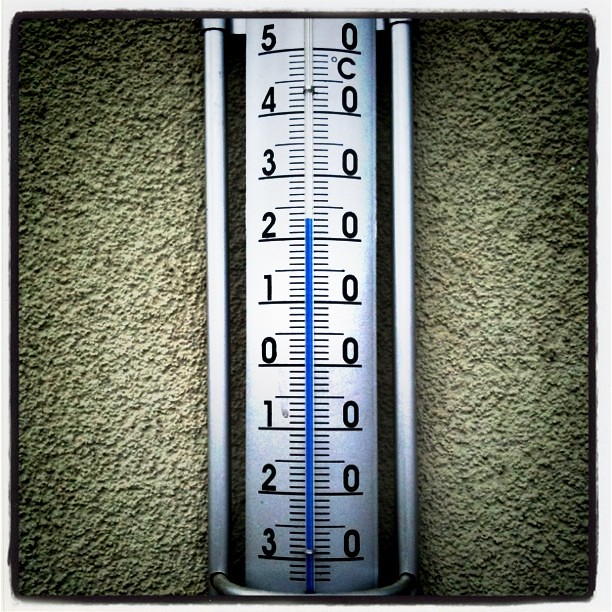The photograph showcases a wall-mounted thermometer set against a deeply textured, cement-like stucco wall. The wall, predominantly gray, features a gradient that transitions from lighter gray at the center to darker shades towards the edges, accentuated by an unnaturally high contrast, likely applied through a filter. The image itself is square-shaped with a thin white border framing it.

The thermometer, situated centrally, is encased in a sleek, thin metal bar that curves around the base and extends vertically along both sides. This tall and narrow instrument is white, featuring a slender blue line indicative of the current temperature. The blue mercury-like substance rises to a level corresponding to approximately 2°C.

On the thermometer scale, the left side numerals sequentially ascend from 0 to 5 as it goes upwards and descend to -3 moving downwards. Conversely, the right side uniformly reads 0, annotated as degrees Celsius at the top. Notably, the blue line extends about three-fifths up the thermometer, surpassing the 2°C mark, illustrating a detailed view of the ambient temperature in the captured moment.